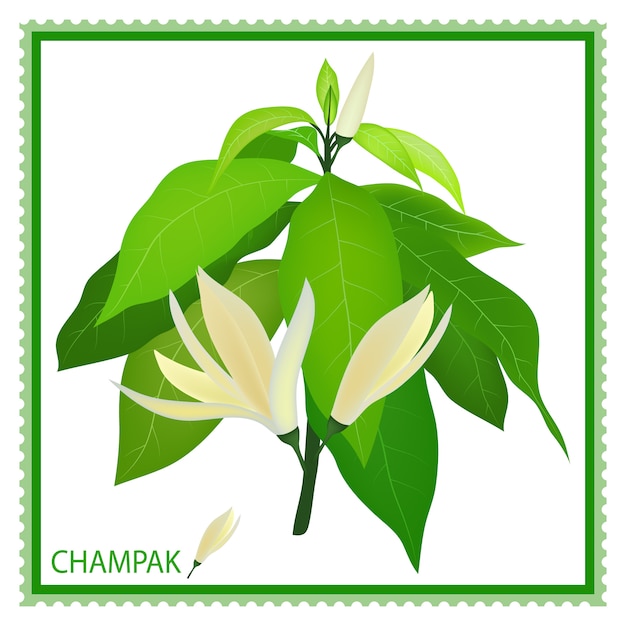The image depicts a square, stamp-like design with perforated edges resembling those of traditional postage stamps. The outer border is a light green, surrounding a darker green interior border. The focal point of the design is a cartoon-style plant with a dark green stem. The plant features an array of leaves: three broad, light green leaves to the left and six to the right, all in a smooth, wide, flat style. At the base of the plant to the right, there is a fully opened fluted white flower with a similar flower situated next to the word “Champak” in the bottom left corner. The word "Champak," spelled C-H-A-M-P-A-K, appears in green font. At the top of the plant, smaller lighter-colored leaves cluster around another fluted white flower, harmonizing with the larger leaves below. The background of the entire design is white, allowing the vibrant greens and whites of the plant and border to stand out distinctly.